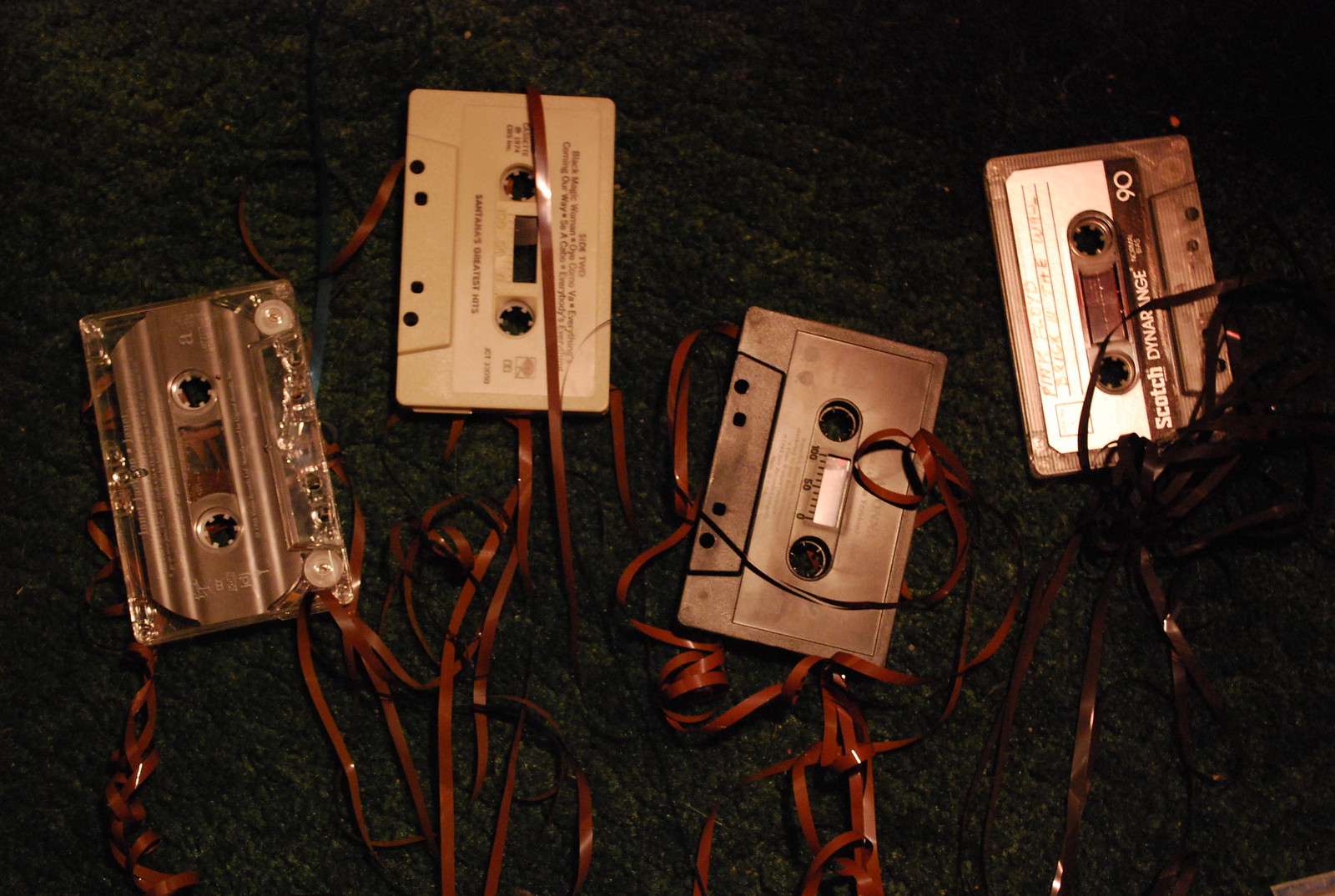This photograph features a nostalgic collection of four cassette tapes lined upright on a table, with their short sides facing the viewer. The cassette tapes are arranged in a staggered formation, with the first and third tapes at the same height, and the second and fourth tapes placed slightly lower. The group consists of three black tapes, one white tape, and a clear tape on the far left. The tapes are tangled with unraveled, dark brown film spilling out, creating a chaotic but aesthetically intriguing scene. Notably, the second tape has a label reading "Santa Anna's Greatest Hits," and the last tape bears the label "Scotch Diner." The scene takes place on a rough, fuzzy blanket or carpet, under the illumination of a single light source, emphasizing the intricate details of the unwound film weaving through and around the tapes.